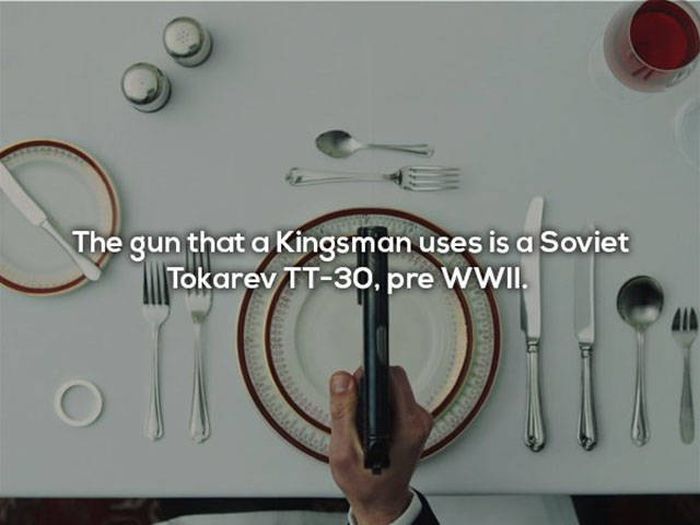The image is a detailed top-down photograph of a dining table set for a meal. The pristine white tablecloth serves as a backdrop for a dramatic scene. At the center, you can see a hand emerging from the bottom of the frame, holding a black handgun aimed upwards. The hand, clad in a white shirt cuff and a black suit jacket, grips the gun firmly. The table is meticulously arranged with a large dinner plate bordered in red and a smaller plate perched on top, both in the center. To the left of this plate are two forks, with a smaller fork above the plate facing right. Positioned to the right of the central plate are two knives, a soup spoon, and a small fork.

In the upper left corner of the table, there are steel salt and pepper shakers. Above the plates, a fork and a spoon are set with their prongs and scoop facing opposite directions, respectively. In the top right corner, a wine glass brimming with a transparent red liquid is visible, adding a splash of color to the otherwise monochromatic setting. A smaller plate with a red rim and a silver butter knife placed on it sits towards the left of the table. 

Text overlaid in the image's center reads, "the gun that a kingman uses is a Soviet Tokarev TT-30 pre-World War II." The text is white with a dark gray outline, creating a stark contrast against the light gray tint of the overall image. The clean, sharp lines of the silverware and the neatness of the table setting juxtaposed with the presence of the firearm create a striking and unsettling atmosphere.